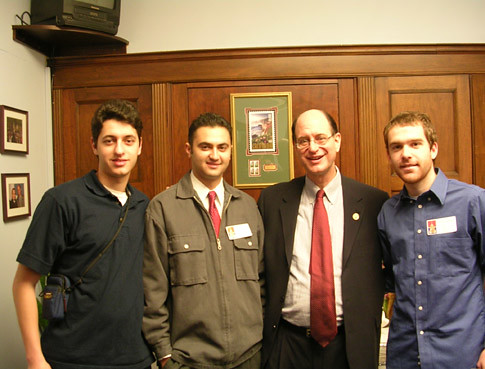This image captures a group of four men posing together in a small, square photograph with no border. They stand against a background consisting of a brown wall, likely doors, with a white wall above it and a small, older-style corner tube TV perched on a brown shelf. The left side of the image shows part of the white wall adorned with a couple of picture frames, one of which is green with a smaller picture inside.

The four men are positioned centrally and appear to be at a formal event, all smiling at the camera. The first man, on the left, wears a navy blue polo shirt and has a belt bag slung over his shoulder; he has short brown hair. Next to him, the second man sports a grey jacket over a white button-down shirt and a red tie, also with short brown hair. The third man, who seems older with a balding head flanked by brown hair, is dressed in a suit with a red tie and white button-down shirt. The last man on the right wears a blue button-down shirt with a name tag on his chest; he too has short brown hair. The overall setting is indoors, characterized by the contrasting hues of white, brown, and various accent colors like green and dark blue.